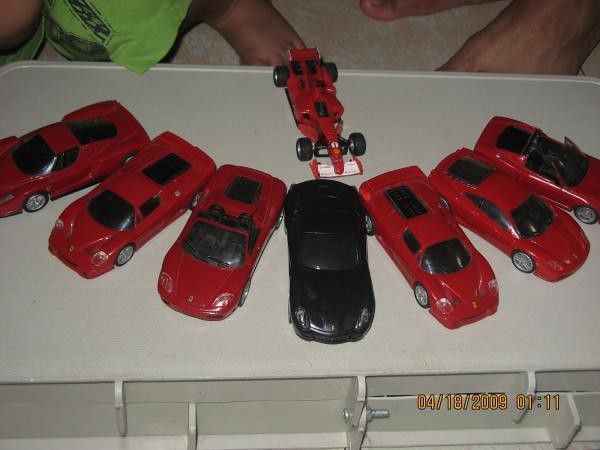The colored photograph, dated 04-18-2009 at 01:11, captures an arrangement of eight toy cars displayed on a white plastic surface, possibly a cooler. At the top of the image, the bare feet of both an adult and a child are partially visible. The toy cars, predominantly red with one black sports car in the middle position, are arranged in a gentle arc from left to right. Most cars resemble sleek, narrow-nosed sports models. The white surface beneath, fitted with a visible hinge near the bottom of the photo, suggests the display is on a hinged lid or cover. The feet in the background hint at a shared moment, possibly a child's pride in their toy collection.